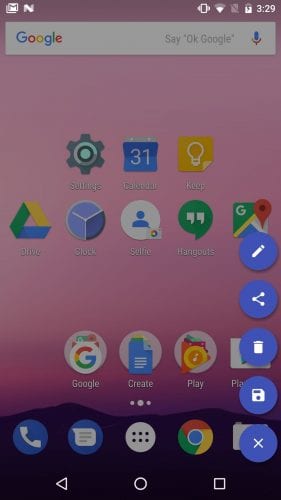A user captured a screenshot of their Android home screen, which we are now viewing in the gallery app. The gallery overlay features options such as Edit, Share, Delete, and Copy. The home screen itself showcases an older version of Android. The backdrop is a scenic sunset with the sun already below the horizon, painting the sky in hues of pink and purple. Silhouetted mountains line the bottom of the screen. The layout suggests a recent installation or reboot, given that many icons are default and grouped in their initial configurations. Key app clusters include Google apps, Play Store services, Calendar, Keep, Settings, Drive, Clock, Hangouts, and Maps. The dock area is home to essential applications such as Phone, Messages, Chrome, and Camera. At the top of the screen, there's a subscription widget labeled "Subscribe."